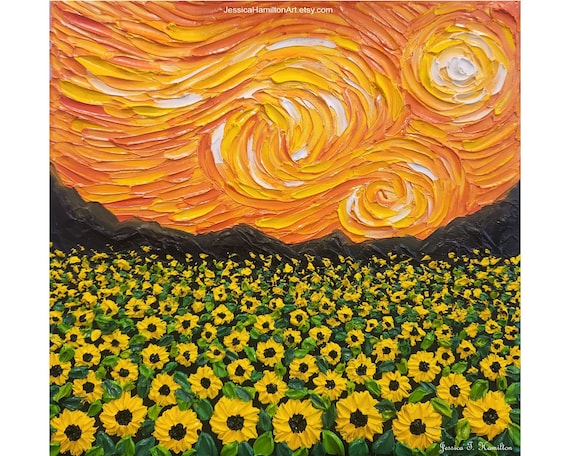A vibrant painting features numerous rows of yellow sunflowers with delicate petals and black centers, surrounded by light and dark green leaves, creating an enchanting foreground. The sunflower field is set against a backdrop of black mountains. Behind the mountains, the sky is painted in rich hues of orange, yellow, and white, resembling a dynamic sunset with swirling brush strokes reminiscent of Vincent van Gogh's "Starry Starry Night." The textured sky, filled with circular, tactile areas, gives a sense of movement and depth. The painting, signed by the artist Jessica J. Hamilton in the bottom right corner, also bears her mark at the top, reading "Jessica Hamilton Art, etsy.com," indicating her authorship. This artwork captivates with its intricate details and rich textures, making it a striking and visually engaging piece.